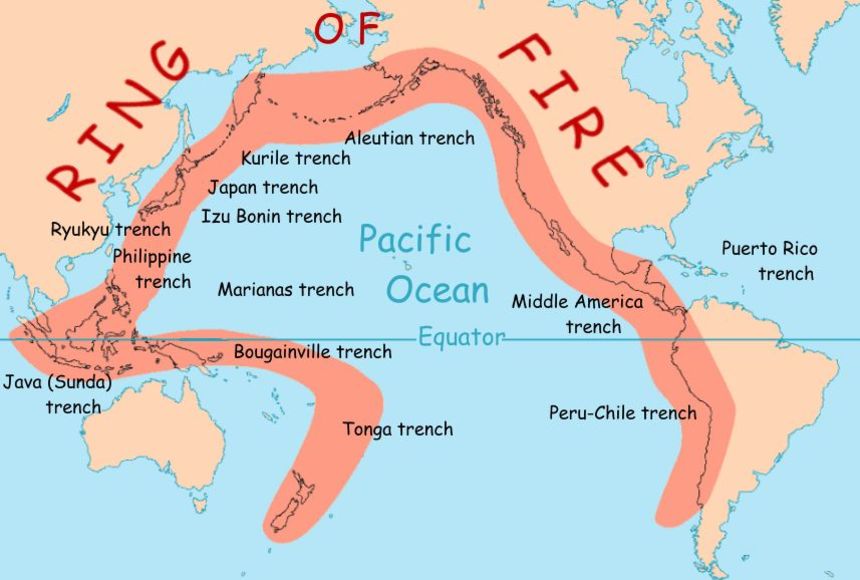This detailed map prominently focuses on the Pacific Ocean, highlighted in a sky-blue hue, with surrounding land masses colored in light beige. It depicts major continents and regions including North America, South America, Australia, Southeast Asia, the Philippines, Indonesia, Japan, Korea, and parts of Russia. The central theme of the map is the "Ring of Fire," which is highlighted in an orange-beige tone along the Pacific Ocean's boundaries. The map outlines the significant volcanic and seismic activity areas, marking the locations of various trenches such as the Middle America Trench, Peru-Chile Trench, Tonga Trench, Philippine Trench, Java Trench, Japan Trench, and Aleutian Trench. The red text at the top clearly labels this ring of intense geological activity as the "Ring of Fire." The highlighted regions trace the volcanic activity zones along the coastal areas of California, Canada, Middle America, and South America, extending through the islands of the Philippines and up to the Bering Strait.